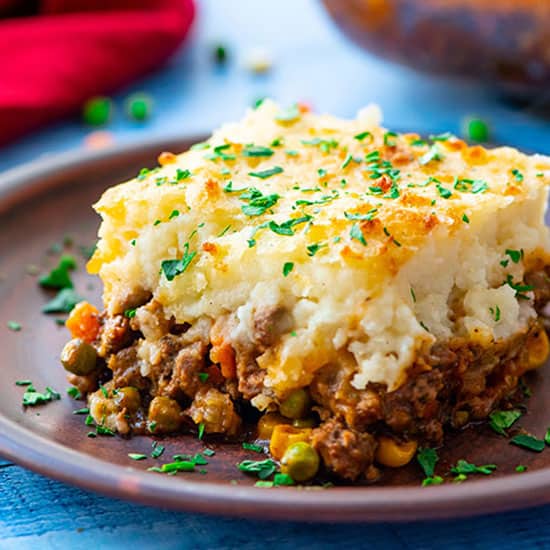The square photograph showcases a meticulously arranged plate of shepherd's pie. The shepherd's pie is richly layered, featuring a hearty base of ground beef interspersed with peas, corn, carrots, and likely a bit of onion. Crowning this savory blend is a generous spread of mashed potatoes, baked to perfection with a golden, crusted top. Delicate green flecks, presumably parsley, are artistically sprinkled across the potato crust, adding a touch of color and garnish, with additional specks artistically scattered around the edge of the dark brown plate. The plate rests on a light blue tablecloth or placemat, adding a soft, contrasting backdrop. For added context, the background of the image reveals a couple of escaped peas and a kernel of corn on the tablecloth, as well as two faintly visible bowls that provide a sense of a complete dining setting.